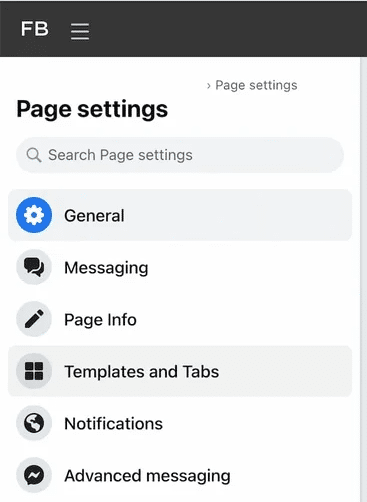The image showcases a website, displayed in a mobile format, likely on a smartphone. The header is a solid black bar featuring the "FB" logo and three horizontally stacked lines, indicating a menu. Below the header, large black letters spell out "Page Settings." Directly beneath this, a light gray, oval-shaped search bar containing a magnifying glass icon prompts users to "Search Page Settings."

Moving further down, the menu is divided into various sections. The first section is labeled "General," accompanied by a small blue circle. Following this is the "Messaging" section, denoted by a gray icon depicting a message bubble. The next section, "Page Info," is marked by a gray circle containing a crayon icon. "Templates and Tabs" come next, identified by a gray circle with a divided square icon in black.

The "Notifications" section features a predominantly black and gray color scheme. Lastly, "Advanced Messaging" is represented by a black icon with a wavy line running through its middle.